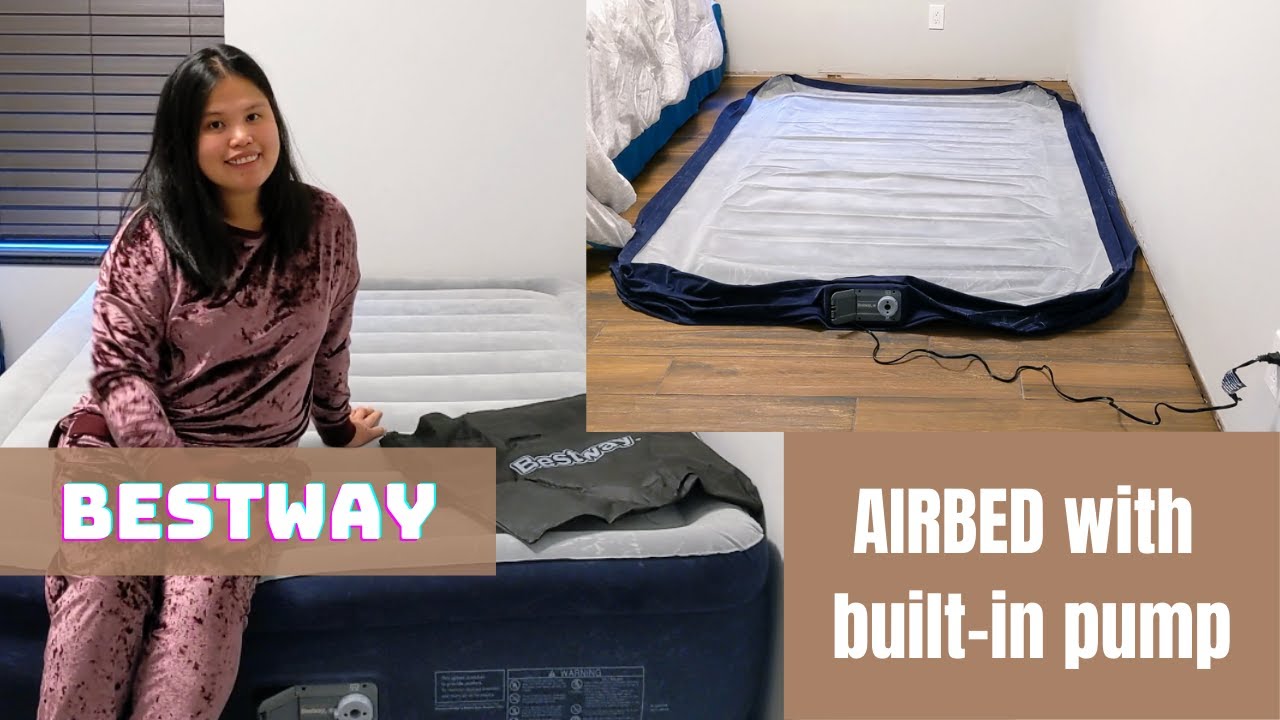The image appears to be an advertisement for an airbed, presented in a landscape layout with two photographs and some text. On the left side, a medium-length black-haired girl, likely a teenager, is sitting on a fully inflated blow-up mattress branded "Best Way." The mattress has a white top and blue sides, with an electric component visible for plugging in the built-in pump. She is wearing a long-sleeve pink velvet outfit and is smiling. The backdrop includes a white wall and possibly a rainy, daylight outdoor setting. The right side of the image shows the same airbed in a deflated state, lying flat on a wood floor with a wire extending to a wall outlet. Above this, there's white text on a brown bar that reads, "airbed with built-in pump." The overall layout suggests the image is designed to highlight the airbed's features and functionality.